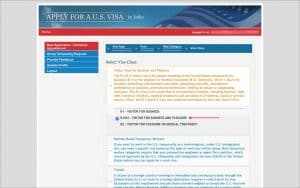This image depicts a screenshot of an official U.S. government website, specifically related to applying for a U.S. visa. The photo is rather small, making it difficult to discern most of the text except for the prominent headers. The image has a landscape orientation, but the elements within the website are arranged in a portrait layout. The photo features gray vertical borders on both the left and right sides, and a thin gray strip along the top.

The header of the website is a vivid blue with a backdrop of the U.S. flag waving gracefully. In bold white letters enclosed with borders at the top and bottom, it reads, "Apply for a U.S. Visa." Below this header, there is a long red horizontal bar featuring white text at the left corner, which is difficult to read, followed by additional white text extending to the right.

Just beneath the red bar, there is some gray space, then a small landscape box situated to the left. This box also has a red header with white lettering. Below this box, there are four narrow, elongated rectangular blue boxes, each with white text.

To the right of these elements, there's a section with a blue header bearing white text, followed by various categories. Positioned below this, there is a black header, the text of which is illegible. This is followed by a long rectangular white box containing yellow text. Further down, there is a gap that includes black text next to a purple pin icon and a red line. This section concludes with two long, narrow white rectangular boxes featuring blue text.

Overall, the website's layout and design elements reflect a formal and official tone consistent with government websites, emphasizing clarity and structure despite some text being unreadable in the small image.